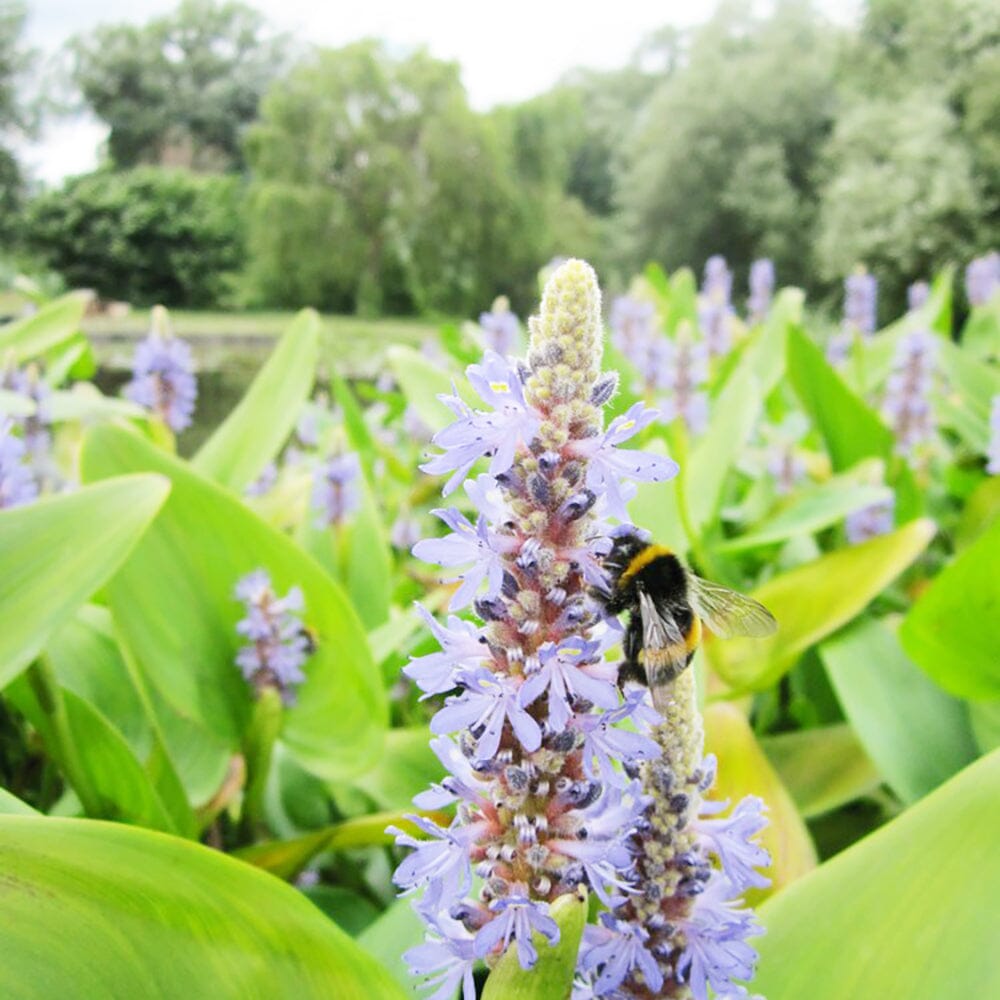A detailed close-up of a bee pollinating a light lavender-colored, stalk-like wildflower nestled among bright green leaves. The bee, centrally positioned in the image, features distinctive transparent wings and yellow and black striping on its body. Its face is buried in the delicate petals of the flower, diligently gathering nectar. Surrounding the main focus, more rows of these delicate flowers can be seen leading to a blurred background filled with greenery, including various trees and bushes. The image's palette prominently features black, yellow, lavender, and green tones, highlighting the vibrant and natural setting.